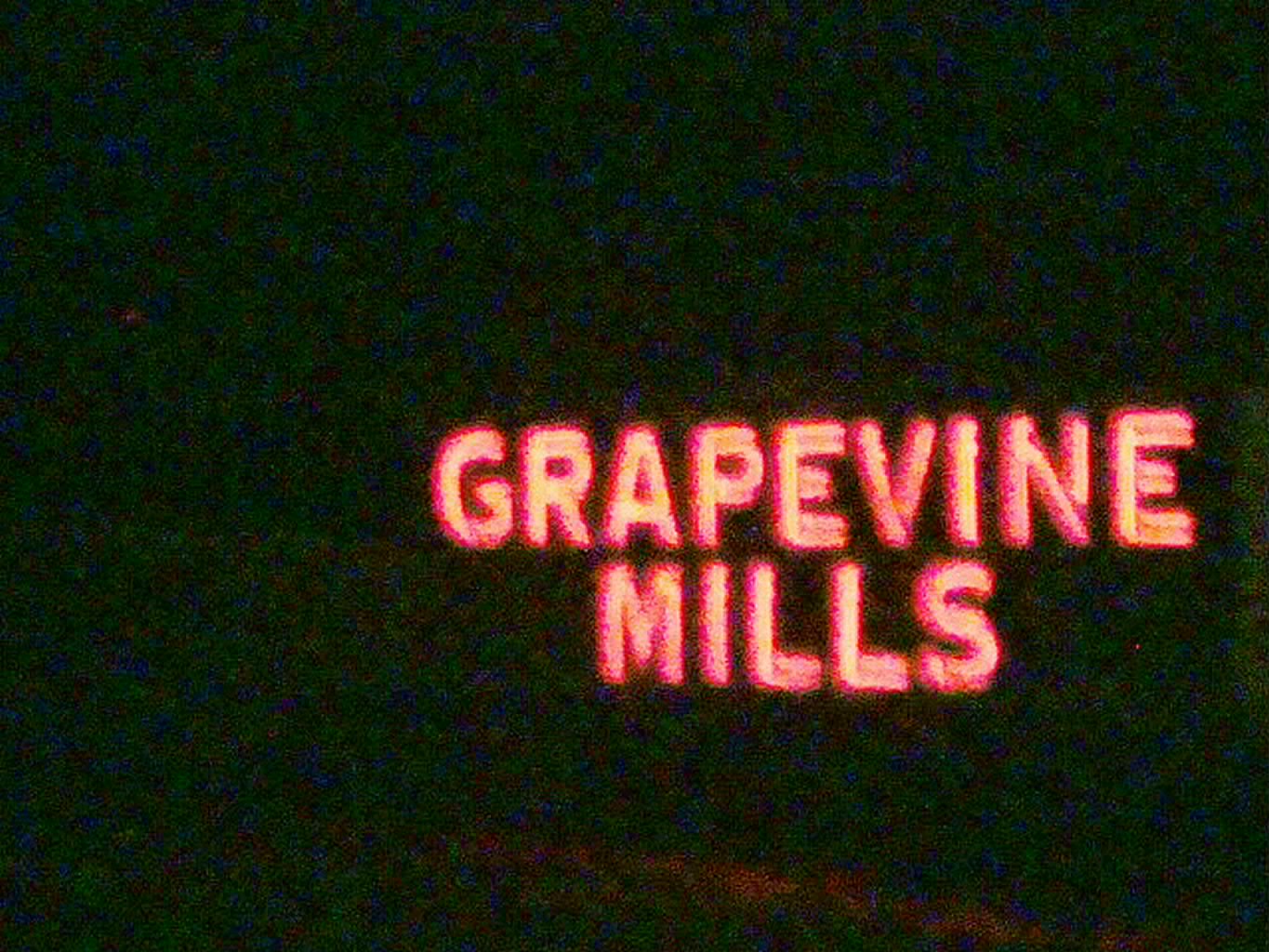In the image, a neon sign displays the words "GRAPEVINE MILLS" in a vivid reddish-orange hue. The sign is split across two lines, with "GRAPEVINE" on the top and "MILLS" directly below it, both in all capital letters. The sign is prominently positioned towards the right side of the composition, close to the bottom right corner. The photo appears grainy, likely taken at night, as the background is pitch black, void of any other details. The neon glow softly illuminates the surrounding area, casting a faint reddish spot on the ground beneath it. The overall effect highlights the sign's prominence and visibility, making it a notable landmark, possibly for drivers or visitors in the area.